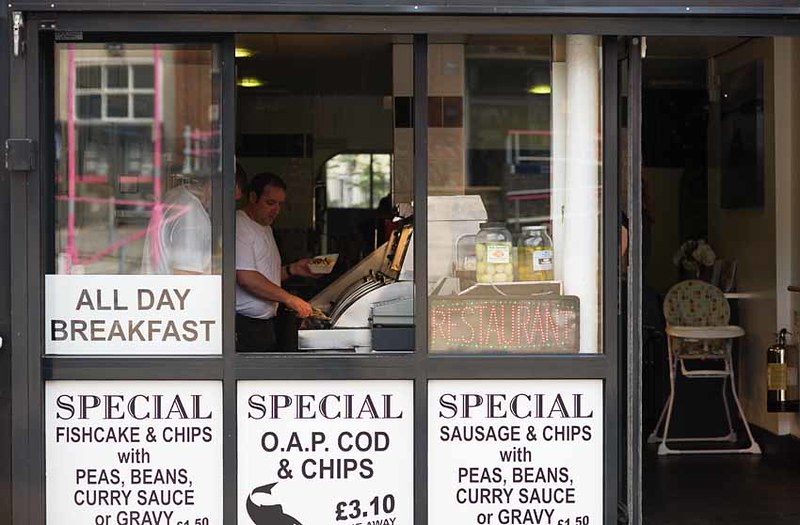This color photograph, captured in landscape orientation, offers an exterior view of a quaint cafe. The facade features six large glass panes arranged in two rows of three, allowing a clear look into the interior. The center top window is open, providing a vivid glimpse of a cashier in profile, wearing a white t-shirt and operating a silver register. 

On the top left pane, a white sign with black text reads "All Day Breakfast." The top right pane showcases a pink chalkboard sign that says "Restaurant." Three signs along the bottom of the windows highlight the day's specials, with text such as "Special Fish Cakes and Chips," and options like peas, beans, curry sauce, or gravy. Prices for these specials vary, including "Special OAP Cod and Chips" for £3.10 and "Special Sausage and Chips" for £1.50.

The black exterior of the cafe contrasts with the bright signage and adds a vintage charm. Reflections of opposite buildings can be seen on the closed left pane. On the right, an open door reveals a high chair facing the viewer, emphasizing the warm, welcoming atmosphere. Behind the counter, mixed among glass jars, and handwritten signs, the cafe scene looks inviting and bustling with activity.